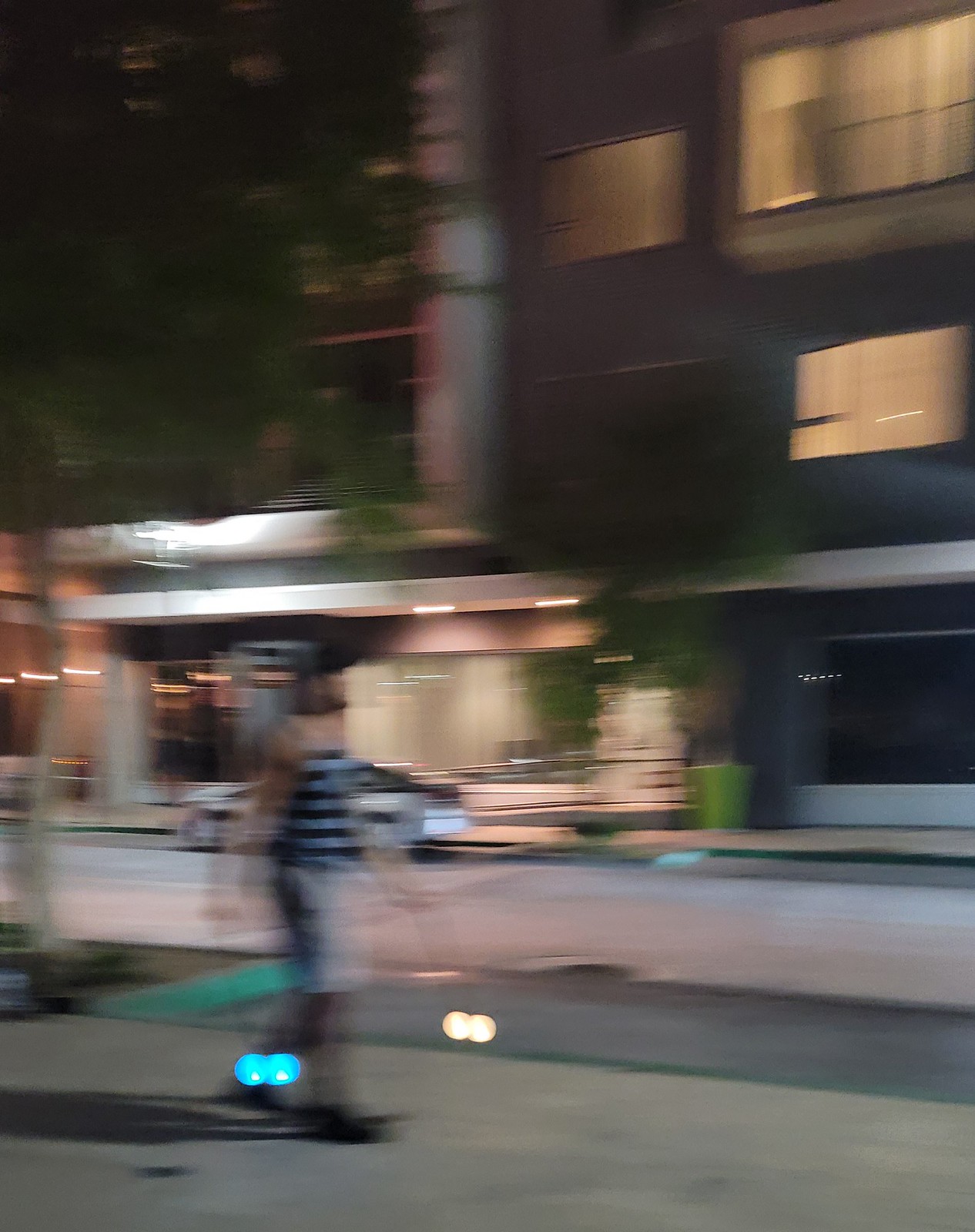This vertically-oriented, low-resolution photograph depicts an apartment building on a dimly-lit street at night. The image captures at least three stories of the building, with a well-illuminated entranceway suggesting a lit lobby behind glass doors. On the sidewalk near the entrance, a person is visible in blurred motion, making their identity indiscernible, but they appear to be wearing a light blue and dark blue striped shirt paired with gray pants. Some rooms on the second and third floors of the building are illuminated, adding more light to the scene. Additionally, a large olive-green planter can be seen outside the lobby doors.